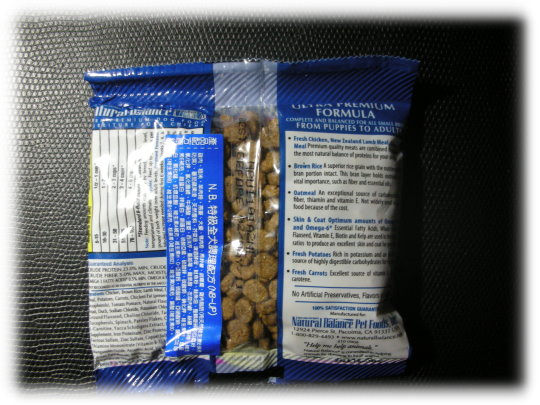The image displays a small plastic package resembling a single-serving portion of dog food kibble. The clear plastic section reveals small, brown, circular pieces that look like dog kibble, and the back of the package confirms this impression. The packaging is primarily medium blue and contains various informative texts, although much of it is difficult to read due to its sideways orientation.

The visible text indicates that the product is labeled as a "premium formula," suitable for "puppies to adults." Ingredients listed include "fresh chicken," potentially "rice" or "oatmeal," and mentions of benefits for "skin and coat." Other ingredients mentioned are "fresh carrots" and "fresh potatoes." Towards the bottom, the text implies that the product is a "natural" option, although specific details are hard to discern.

An image of the kibble is displayed on the package, accompanied by some writing in an Asian script, which further adds to the complexity of reading the label clearly. Additionally, some text appears upside down, contributing to the difficulty in fully understanding the package's information.